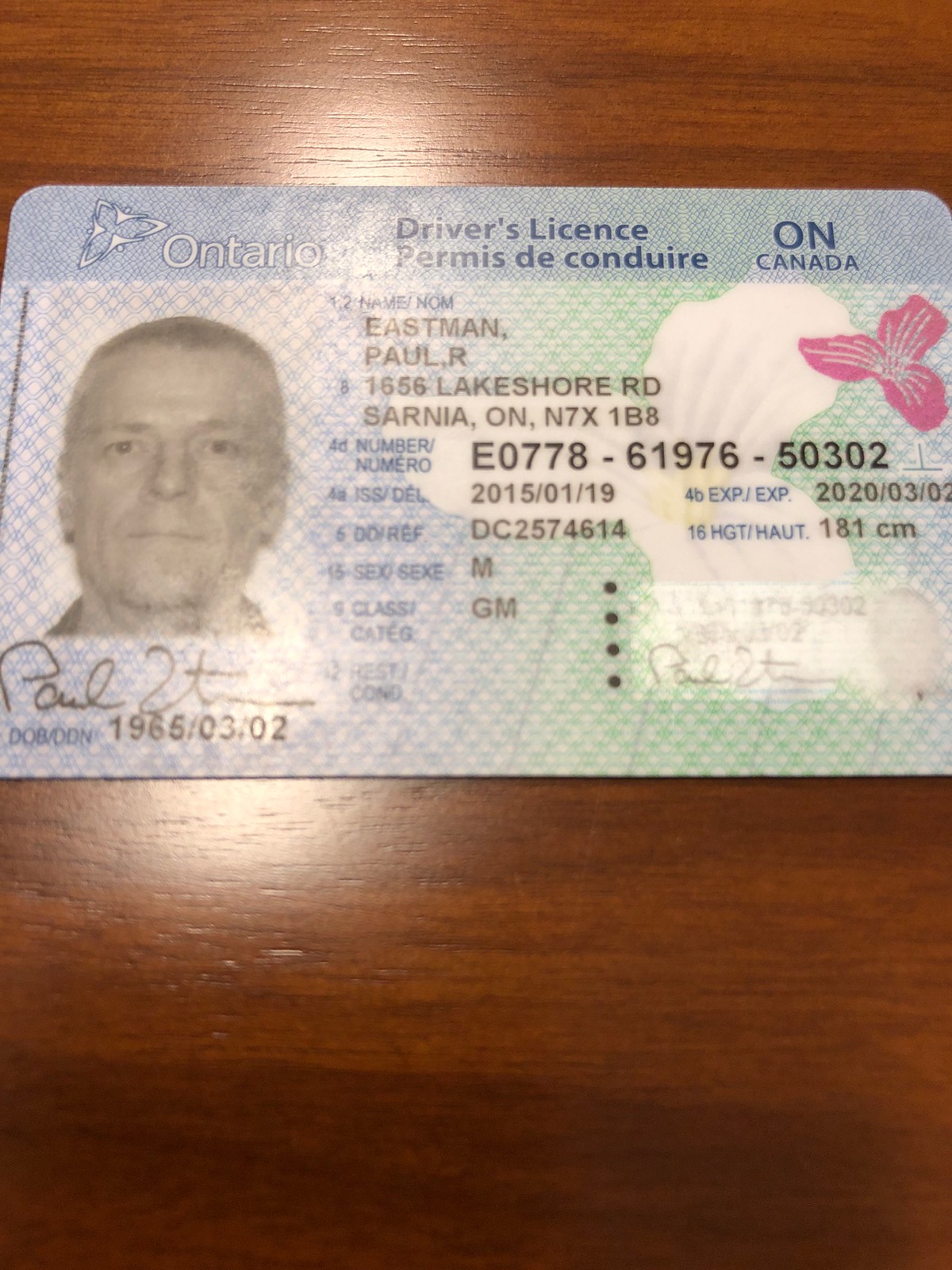This image features an Ontario driver's license belonging to Mr. Paul R. Eastman. The driver's license has a blue and green background with a pink flower logo in the upper right corner. The top of the license reads "Ontario Driver's License" and "Permis de Condoire." Paul's personal details are clearly shown, including his address: 1656 Lakeshore Road, Sarnia, Ontario, N7X 1B8, sex: male, and date of birth: March 2, 1965. The document was issued on January 19, 2015, and it expires on March 2, 2020. A black and white photo of Paul is located on the left side of the license, depicting him as an older man with short, likely grey hair. His signature is positioned below the photo. Additional details on the license include a reference number, his licensing class labeled as GM, and his height. The overall layout and identifying marks such as the white and red flower logos contribute to the document's official appearance.